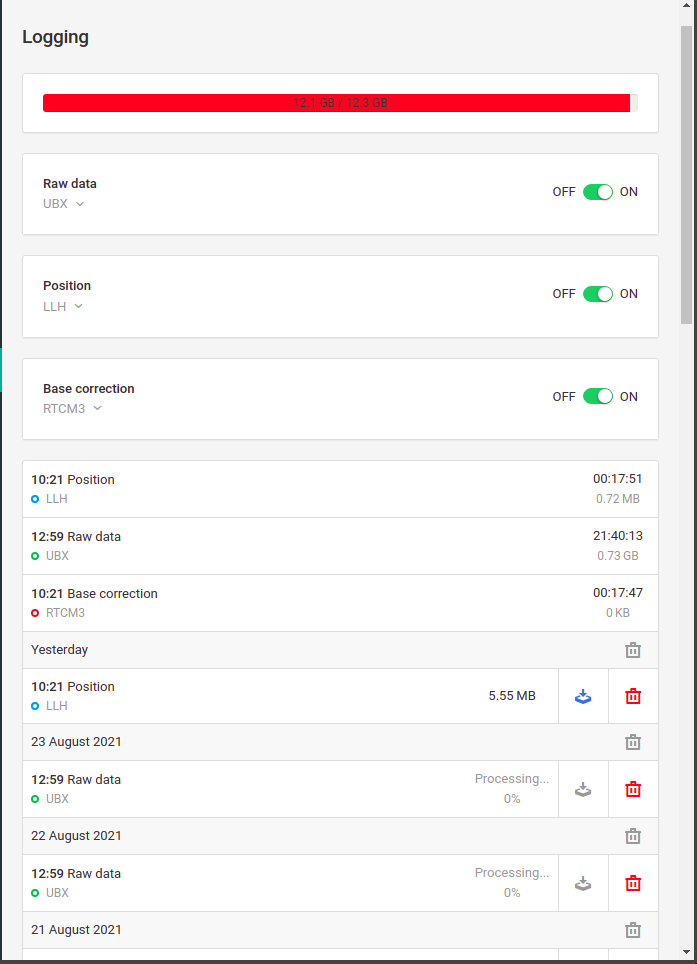This is a detailed description of a report page screenshot displayed on a computer screen. The page has a light gray background and is organized into several sections, each defined by a white rectangle bordered with a thin medium gray line.

At the top left of the screen, "Logging" is prominently displayed in black text. 

The first section features a nearly full red progress bar with a small light gray segment remaining on the right. Overlaid on the progress bar in black text, it reads "12.1 gigabytes / 12.3 gigabytes."

In the second section, on the left side in bold, black text, it says "Raw Data." Below this, in lighter text, it reads "UBX" with a downward-pointing arrow. On the right side of this section, there is an active selection button. The button is green on the left and has a white circle on the right; labels indicate "Off" on the left and "On" on the right, with the button set to "On."

The section beneath this also has a similar selection button to the right, currently toggled to "On." On the left, it reads "Position, LLH," with an arrow pointing downwards.

The following section is labeled "Base Correction" in bold black text with "RTCM3" beneath it in lighter text and an arrow pointing downwards. On the right side, there is another identical selection button toggled to "On."

The next, fairly large section is divided into various rows. The first three rows have white backgrounds with bold text at the top of each. The first row is labeled "10.21 Position" with light text "LLH" beneath it. The second row reads "12.59 Raw Data" followed by "UBX" in lighter text. The third row displays "10.21 Base Correction" with "RTCM3" beneath it. Each of these rows has a colored donut shape to the left of the light gray text in the second row: the first donut is blue, the second is green, and the third is red. There are additional details to the right of each colored donut, and more rows continue below this described portion.